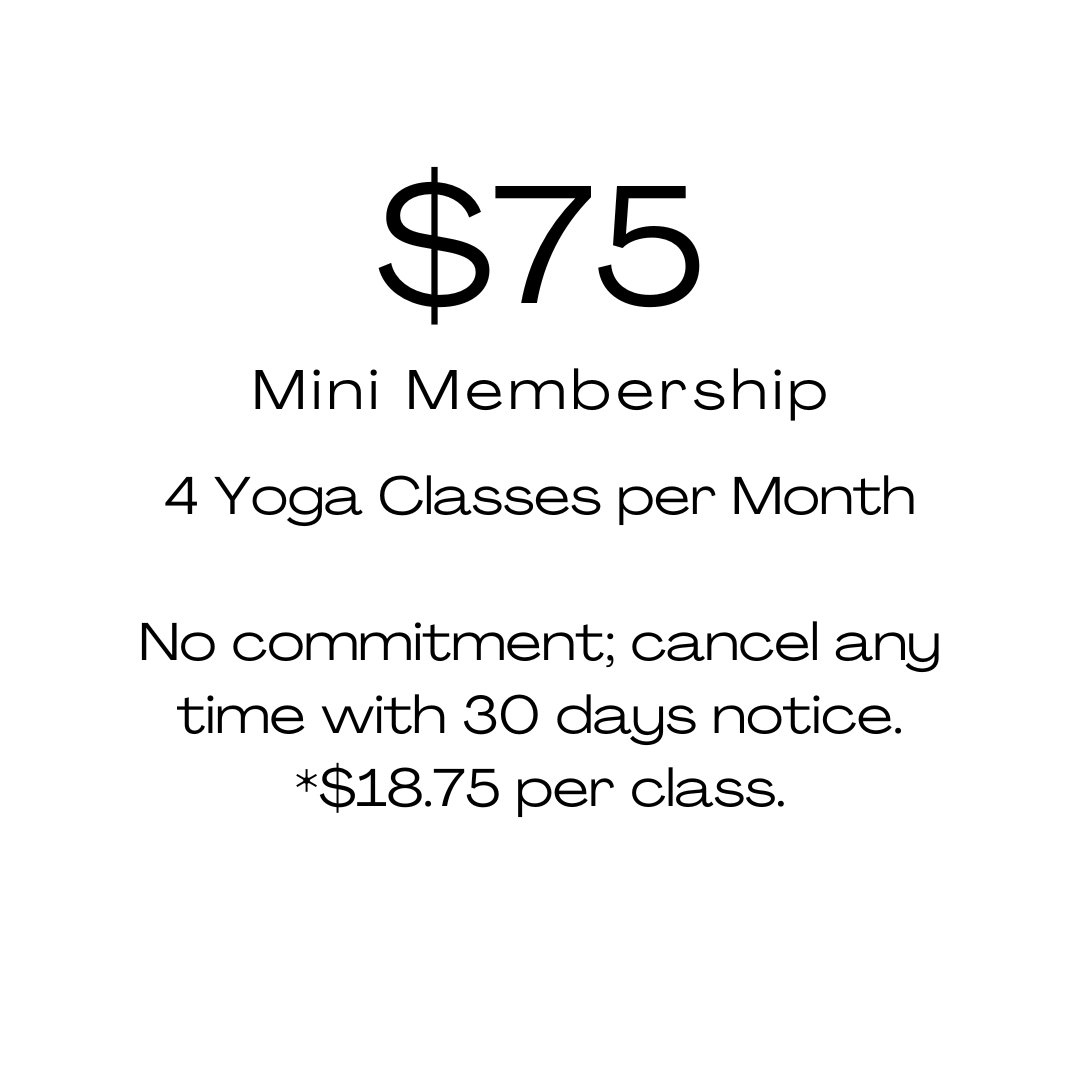Here is a cleaned-up and detailed descriptive caption for the image:

---

The image features a minimalistic advertisement for a membership package at a gym or yoga studio. The design is set against a pure white background, creating a clean and modern look. At the top center, in large black sans-serif font, the price "$75" stands out prominently. Below this, the offer is detailed in five lines of smaller black sans-serif text, also center-aligned. 

The first line reads "Mini-Membership," followed by the second line which states "Four Yoga Classes per Month." 

There is a noticeable gap before the next set of text, emphasizing the key benefits of the membership. The third line at the bottom section reads, "No commitment, cancel any," while the fourth line continues with "time with 30 days notice." The very bottom line, marked with an asterisk, clarifies the cost per class: "$18.75 per class." 

The text arrangement forms an hourglass shape, starting narrow at the top with "$75," expanding slightly with the membership details, and then tapering back in towards the bottom. The overall design is simple and straightforward, effectively communicating the offer for yoga classes in a visually appealing manner.